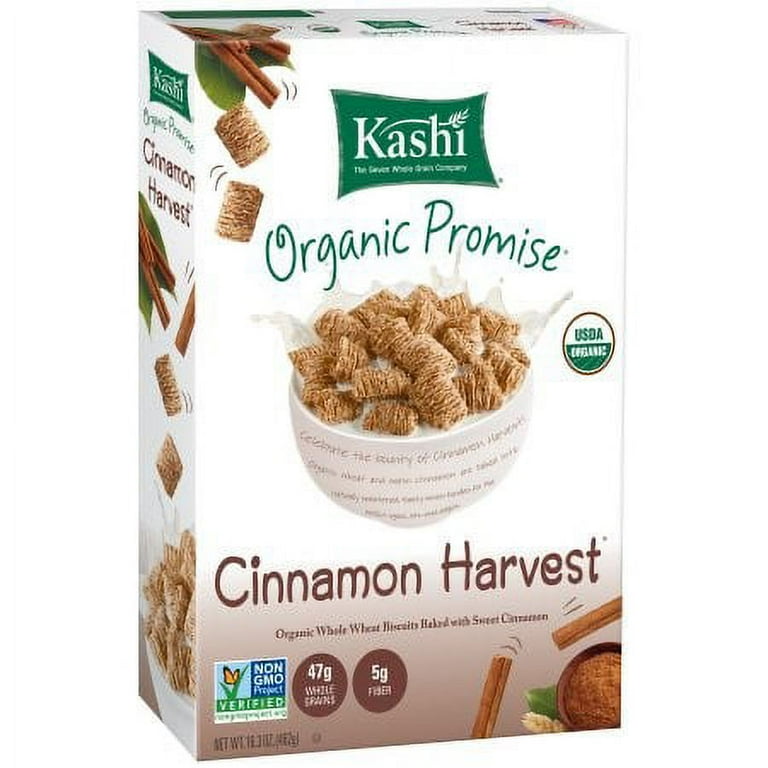This is a commercial-style image of a Kashi Organic Promise USDA Organic Cinnamon Harvest cereal box taken from a three-quarter view. The product features organic whole wheat biscuits baked with sweet cinnamon. The label prominently displays certifications, like USDA Organic and Non-GMO Verified, and nutritional information including fiber content. The box, designed with attractive colors—green, white, wheat, brown, and blue—also includes images of cinnamon sticks. The setting is minimalist with a white background, emphasizing the product, possibly suited for an Amazon or grocery store listing.